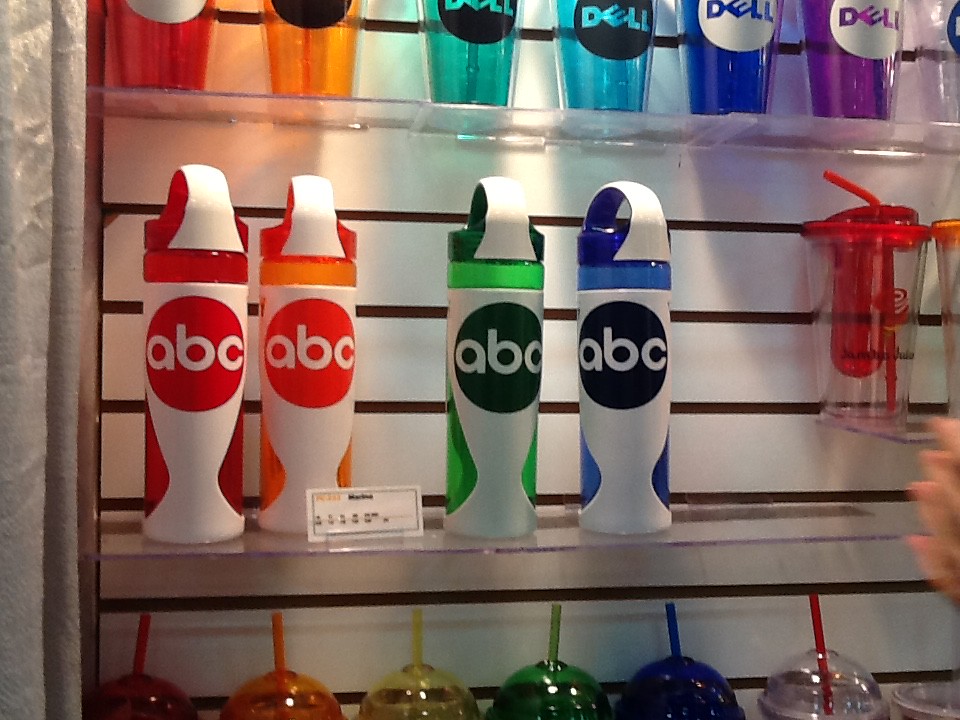The image depicts a store display featuring various plastic water bottles meticulously arranged on clear acrylic shelves against a white grid wall designed with gaps for adjustable shelving. Central to the composition is a middle acrylic shelf, prominently showcasing four identical reusable water bottles distinguished only by their color accents. Each bottle features a white body with a handle-integrated lid and a translucent section in red, orange, green, and blue hues respectively. All the bottles bear a circle emblem with the letters "ABC." Above these bottles, the top shelf displays six translucent cups in rainbow colors, each emblazoned with the Dell logo, and beneath them, partially visible, is a lower shelf holding cups with dome lids and straws in an array of colors: red, orange, yellow, green, blue, and clear. A silver frame adjacent to the grid wall adds a finishing touch to the well-organized storefront display.